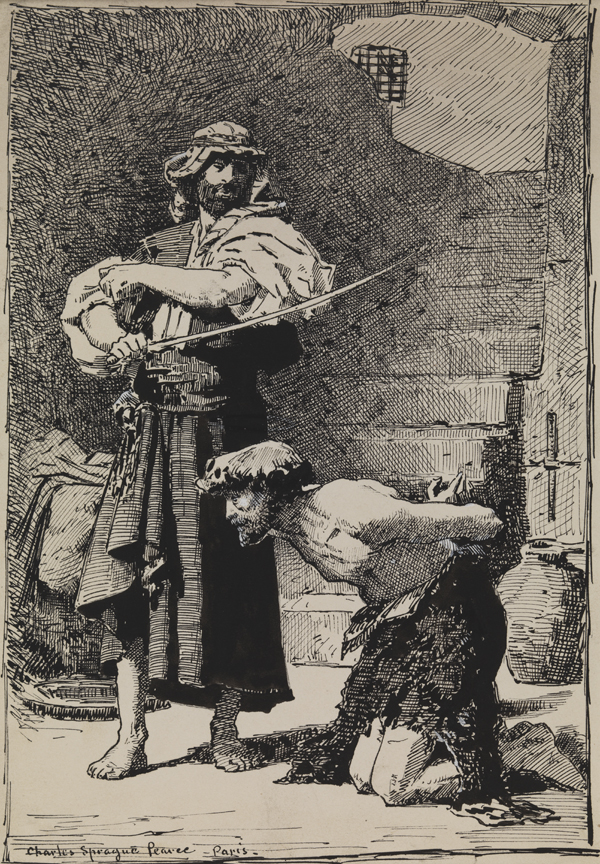This striking black-and-white sketch, in vertical portrait orientation, depicts an intense and historical scene potentially representing the decapitation of John the Baptist. At the center-right towards the bottom, a shirtless man in tattered clothing kneels with his arms bound behind his back, bent forward in submission. The executioner stands above him, poised to strike with a sword. He wears robes and rolls up his sleeves, suggesting preparedness for the grim task. Both men are set against a sketchy backdrop featuring a stairway and a wall, with a large ornate urn to the right. The artist, Charles Sprague-Pierce-Aparis, has signed the illustration at the bottom left corner. The detailed sketch style and the absence of color other than shades of black, white, and gray, emphasize the somber and dramatic nature of the scene.